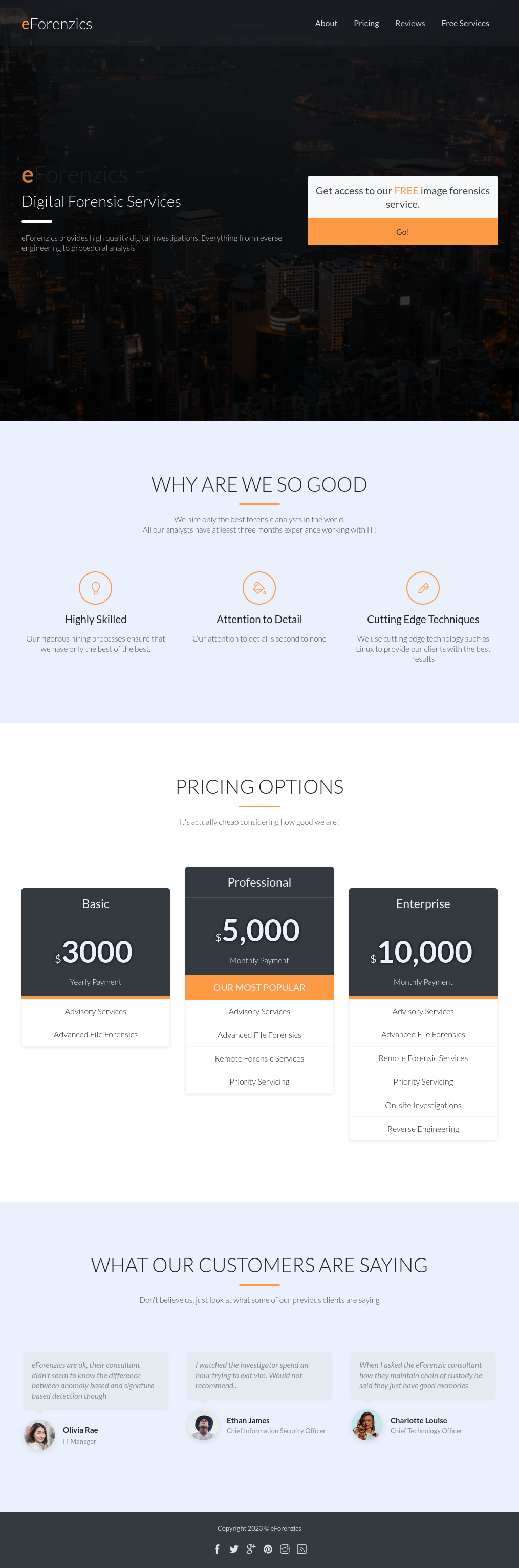Screenshot of the Homepage of East Forensics Website:

The screenshot captures the homepage of East Forensics, a website offering digital forensic services. The overall aesthetic is dark and black, giving it a sleek yet mysterious appearance. The image quality is clear, but the screenshot is taken from a distance, making it slightly harder to read smaller text.

- **Top Left**: The header prominently displays "Digital Forensic Services". Below it, a tagline reads, "East Forensics provides high-quality digital investigations, everything from reverse engineering to procedural analysis."

- **Top Right**: There is a call-to-action button that says, "Get access to our free image forensic services" with a "Go" button beside it.

- **Main Content**: The central part of the homepage features a question, "Why are we so good?" followed by a brief statement: "We hire only the best forensic analysts in the world. All our analysts have at least three months experience." (Note: There is a minor typo in "experience" which is spelled as "experienc.")

- **Highlights Section**: 
  - **Highly Skilled**: Accompanied by an icon of a light bulb.
  - **Attention to Detail**: Represented by an icon of a paint bucket with a ripple effect above it.
  - **Cutting Edge Techniques**: Illustrated with an icon of a pen.

- **Pricing Options**: 
  - **Basic**: $3000
  - **Professional**: $5000
  - **Enterprise**: $10,000
  The pricing section emphasizes affordability despite the high-quality services offered.

The design and information presented on this homepage aim to establish credibility and attract potential clients seeking expert digital forensic analysis.